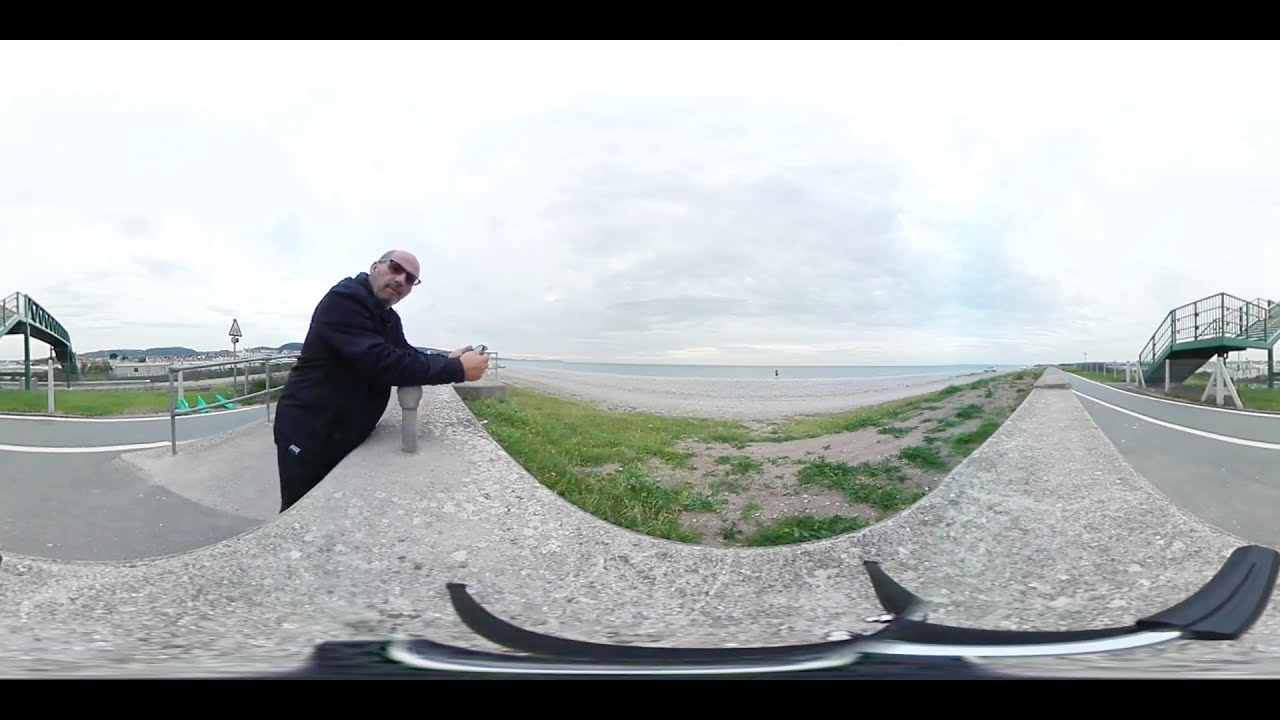In the foreground of the daytime outdoor image, a man dressed in a black long-sleeved shirt, black pants, and sunglasses is leaning against a waist-height stone wall, seemingly looking either at his phone or towards the camera. This scene is set against a distorted backdrop, creating an unusual perspective that makes it appear like two images merged together. Behind the man stretches a view of the beach with its sand, shoreline, and the ocean under an overcast sky. To the right, an outdoor pathway is visible, leading up to green stairs with a green fence, which ascend to an elevated platform. There's also an asphalt road and what seems to be parking and additional walkways in the background, with buildings in the distance. This unusual perspective gives the image a slightly surreal quality, particularly at the edges where it appears curved and not true to life.